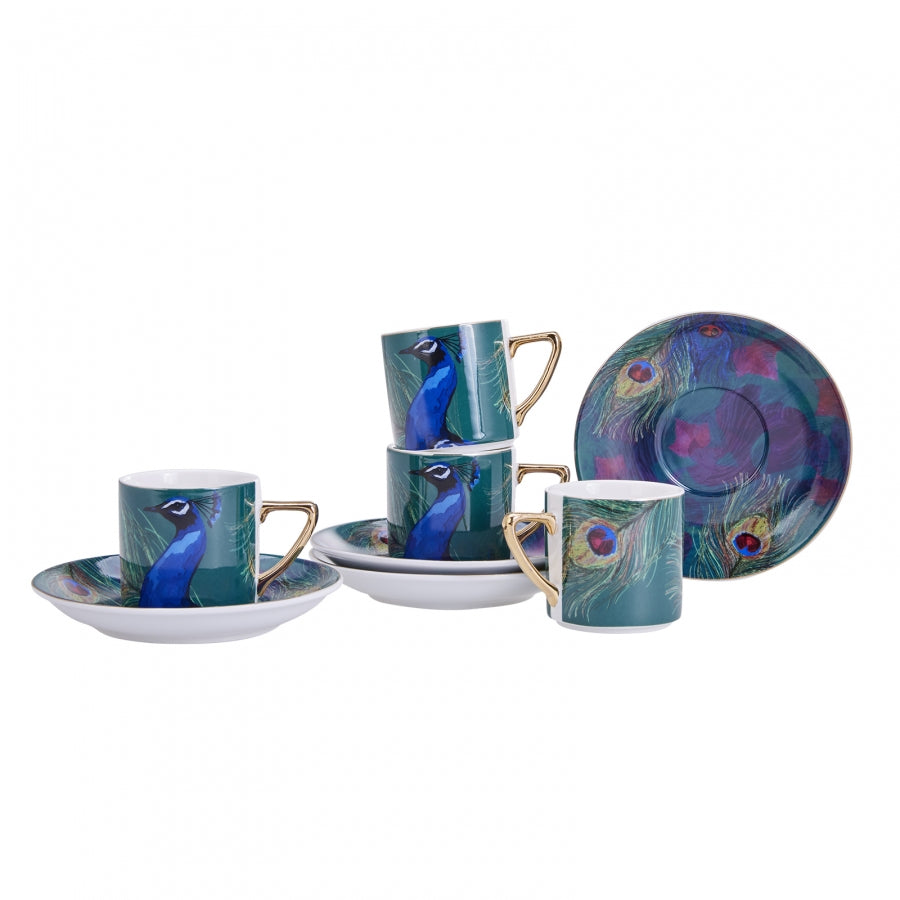The image features an elegant display of hand-painted teacups and saucers, set against a white background, likely a kitchen or showroom. There are a total of four mugs and four saucers. Each mug is adorned with a vivid blue peacock, detailed with a dark blue neck, a light blue chest, and a black beak with white lining around the eyes. The handles of the mugs are shaped like half a 'V' and are gold in color, adding a touch of opulence. Three of the mugs, which showcase the same peacock design, are placed on their respective saucers; two of these mugs are stacked on top of each other. The fourth mug, turned to display the back, reveals a colorful leaf design composed of blue, red, and yellow, matching the vibrant detailing seen on the plates. The saucers, two of which are visible from the bottom, also feature consistent floral and leaf patterns with hues of purple, teal, green, and flat greens. The meticulous design and arrangement highlight the artistic quality of the set, emphasizing the intricate peacock and floral motifs.